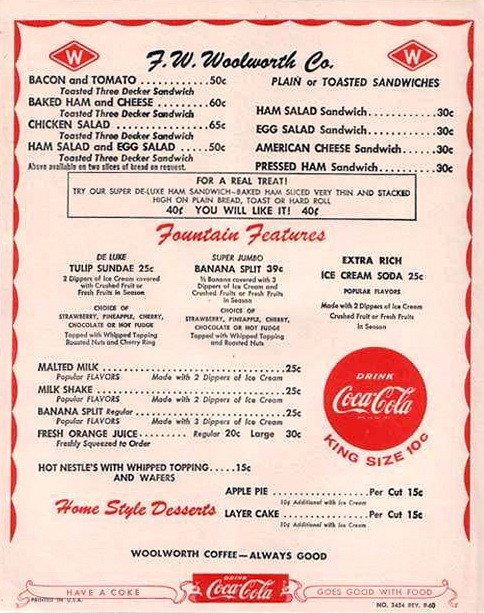This image showcases a vintage menu from FW Woolworth Co., featuring a salmon-colored background adorned with a red banner at the top. The header, written in black font, prominently displays "FW Woolworth Co." directly below it, the menu offers a selection of "Plain or Toasted Sandwiches," including:

- Bacon and Tomato: 50 cents
- Baked Ham and Cheese: 60 cents
- Chicken Salad: 65 cents
- Ham Salad and Egg Salad Combo: 50 cents
- Ham Salad Sandwich: 30 cents
- Egg Salad Sandwich: 30 cents
- American Cheese Sandwich: 30 cents
- Pressed Ham Sandwich: 30 cents

For a special treat, the menu suggests their "Super Deluxe Ham Sandwich" featuring baked ham sliced thin and stacked high on plain bread, toast, or hand roll for 40 cents.

The "Fountain Features" section includes:

- Deluxe Tulip Sundae: 25 cents
- Super Jumbo Banana Split: 39 cents
- Extra-Rich Ice Cream Soda: 25 cents (available in popular flavors made with two scoops of ice cream, crushed fruit, or fresh fruits in season)
- Malted Milk: 25 cents
- Milkshake: 25 cents
- Banana Split: 25 cents
- Fresh Orange Juice (Regular): 20 cents (Large): 30 cents (freshly squeezed to order)
- Hot Nelly's with Whipped Topping: 15 cents
- Apple Pie (per cut): 15 cents
- Layer Cake (per cut): 15 cents

The menu also highlights "Home-style Desserts" in red font and finishes with "Woolworth Coffee, Always Good." At the very bottom of the image, banners on either side of the Coca-Cola logo proclaim "Coke Goes With Food."